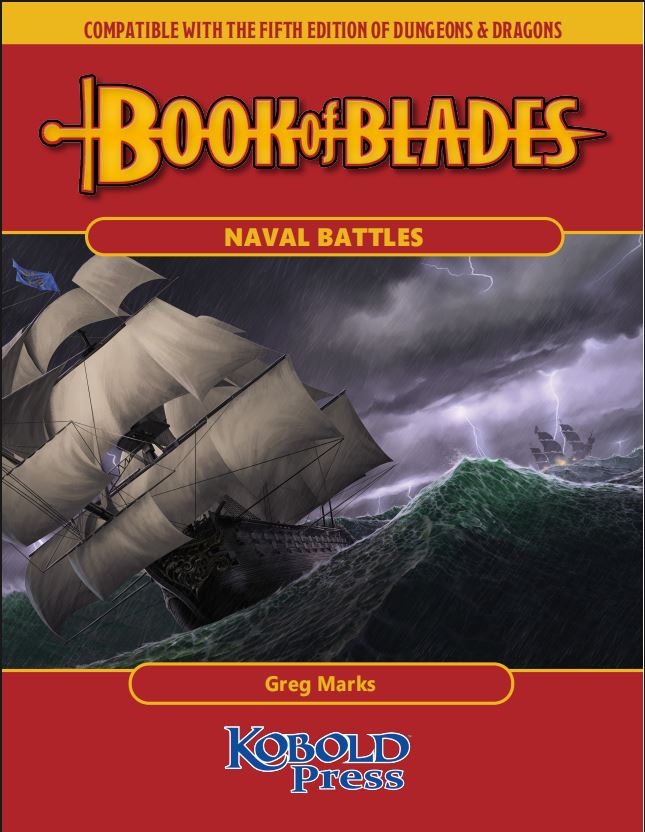This detailed image serves as the front cover of an advertisement for a new study module titled "Book of Blades: Naval Battles," compatible with the fifth edition of Dungeons & Dragons. The prominent design features a dramatic scene where clipper ships navigate treacherous seas under a stormy sky filled with lightning and dark clouds. Large waves crash around the ships, adding to the chaotic atmosphere. Central to the cover is a vibrant and bold color palette, including reds, yellows, forest greens, blues, electric whites, grays, blacks, and browns, that vividly bring the scene to life.

At the top of the cover is a gold bar with red text declaring, "Compatible with the 5th Edition of Dungeons & Dragons." Below this slogan, bold yellow letters framed by a sword design spell out "Book of Blades." Further down, the words "Naval Battles" are prominently displayed, linking to the book's theme. The author, Greg Marks, is mentioned at the bottom in blue text next to the name of the publisher, Kobold Press. The outdoor setting and dramatic imagery perfectly encapsulate the intense and adventurous naval warfare scenarios this Dungeons & Dragons module aims to explore.